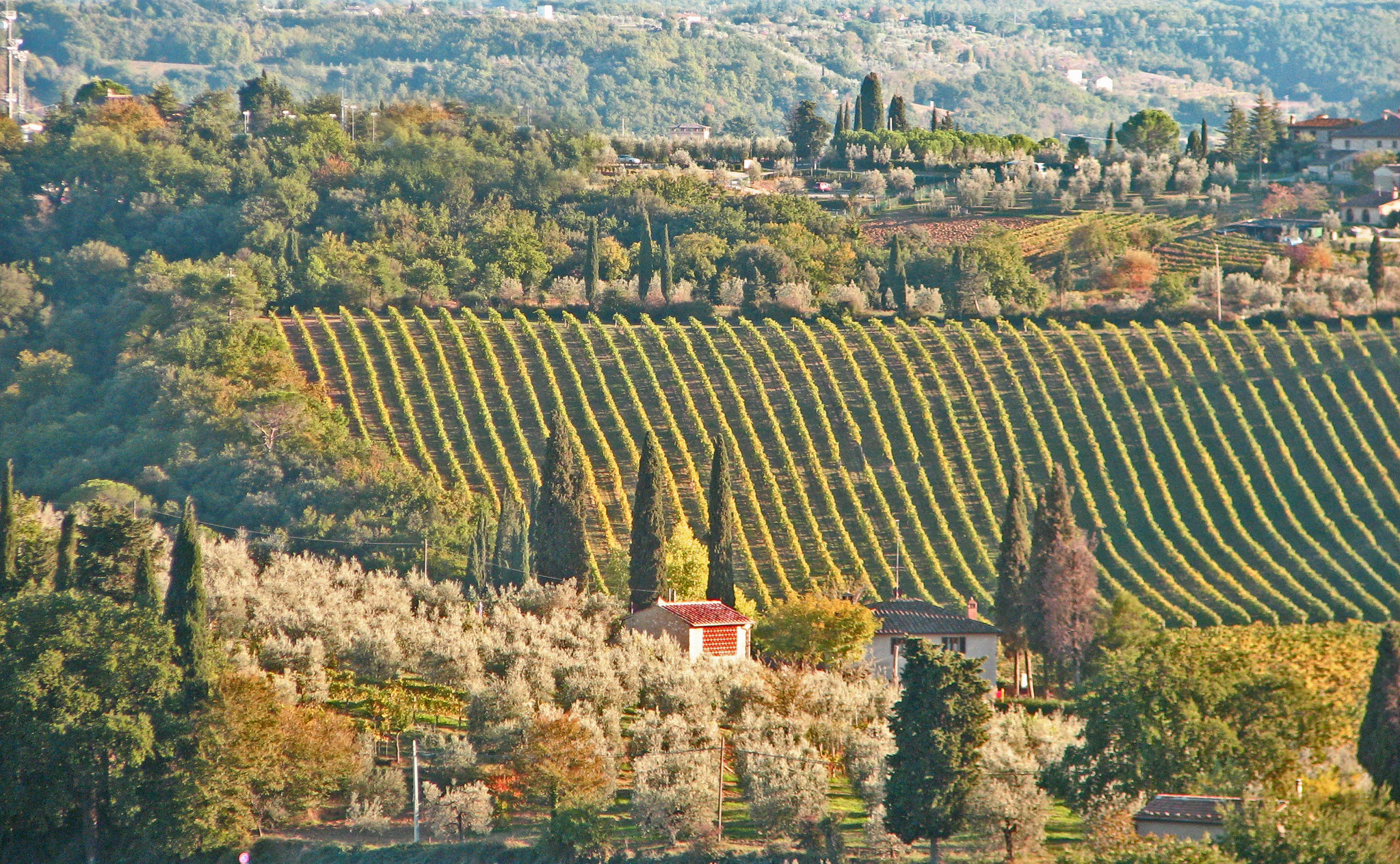The photograph captures a stunning outdoor landscape, taken from an elevated vantage point such as a hilltop, overlooking a vast expanse of meticulously maintained farmland. The central part of the image features extensive fields, distinguished by neatly aligned rows of bright green crops, possibly a vineyard, with noticeable gaps between each row, suggesting the plants are several feet tall. Interspersed among the fields are a diverse array of trees; some adorned with white flowers, others evergreen, adding a variety of colors and textures to the scene.

In the foreground, towards the lower section of the photograph, there are two small buildings—one with a white facade and flat roof, and the other smaller with a brown roof. These structures, likely homes, are nestled among the trees, which include spear-shaped Italian cypress, characteristic of the Italian countryside. The edges of the fields are bordered by a wooded area that curves from the left side of the image.

Beyond the cultivated fields, the landscape transitions into higher hills or possibly mountains, partially obscured at the top edge of the photograph, giving a sense of depth and distance. The background is slightly hazy, filled with a mix of vegetation and sporadic homes, enhancing the rustic charm of this picturesque countryside.